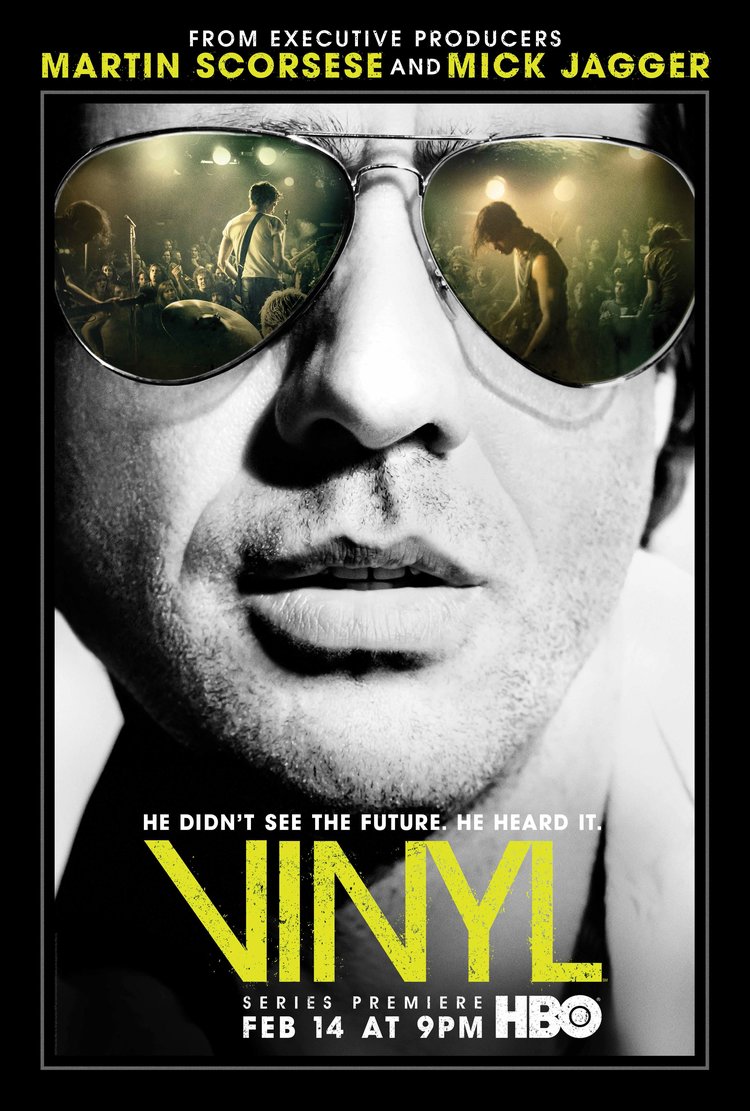On a stark black background is a striking movie poster. At the top, white text reads, "From executive producers Martin Scorsese and Mick Jagger." Dominating the center is the face of a gentleman, characterized by his scruffy close-cut beard and reflective sunglasses. In the reflective lenses, we see a vibrant indoor club scene, featuring a band of four male musicians performing energetically. One of the musicians has a guitar strap visible across his back, and the neck of a guitar juts upward from the left lens. Beneath the man's face, white text reads, "He didn't see the future. He heard it." In large, bold yellow letters, the title "Vinyl" stands out prominently. Further details in sizeable yellow fonts announce, "Series Premiere February 14 at 9 p.m. on HBO," with "HBO" rendered in notably large white letters.